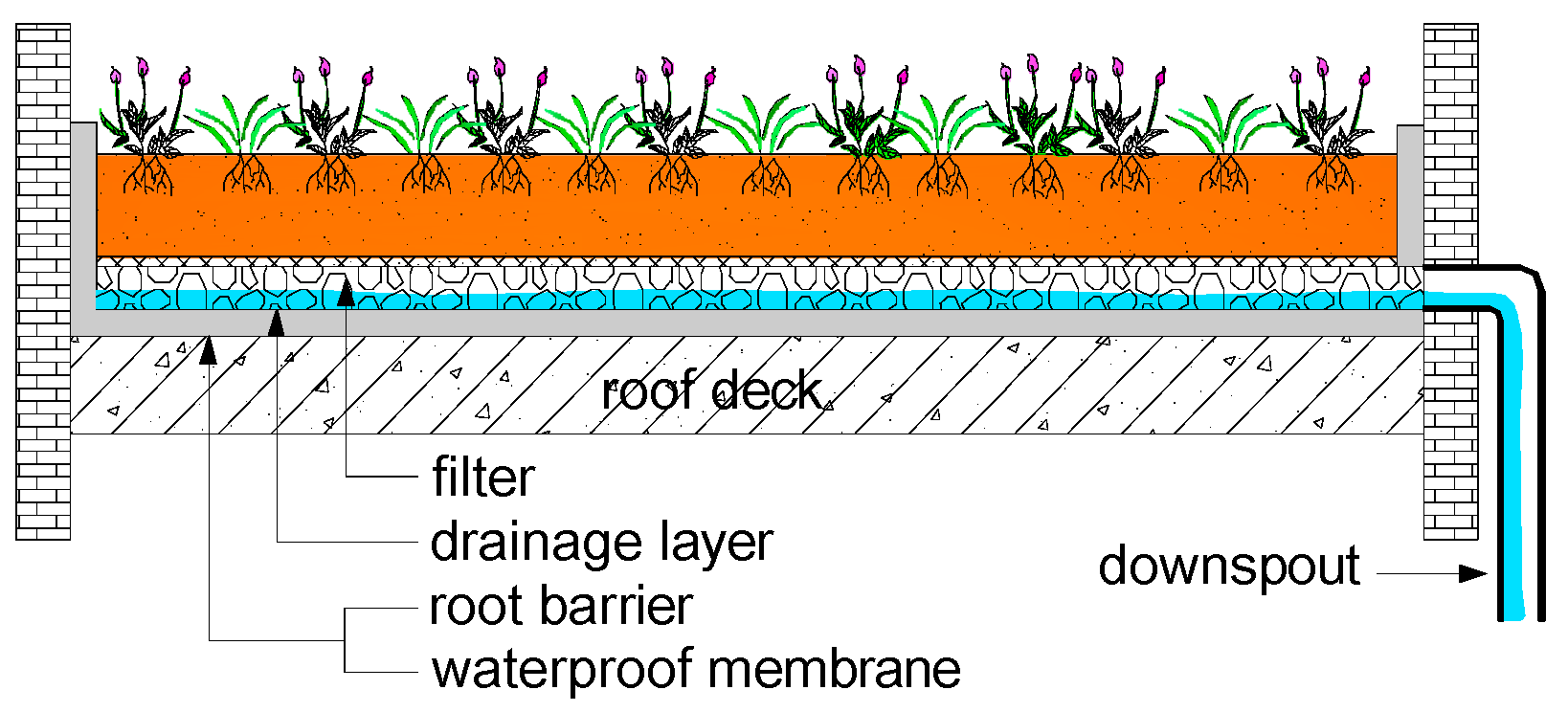This image is a detailed, horizontally-aligned diagram illustrating a rooftop garden infrastructure. On the far left and right sides, there are vertical, black-and-white brick columns. Between these columns, at the top of the image, there is a thick, horizontal, orange rectangle covered with tiny black speckles, representing soil. Growing from the soil are multiple sets of plants with black roots and stems. These plants have bright green leaves and small clusters of purple flowers with about eight clusters spaced evenly across the image.

Below the soil layer is a detailed depiction of various layers crucial for plant growth and infrastructure stability. Directly beneath the orange soil layer is a black-and-white section illustrating small rocks, some of which are shaded in blue, likely representing water. Below this rocky area is another horizontal rectangle with diagonal lines labeled "roof deck."

The depiction also includes annotations pointing to different parts of the image. These annotations label the sections as follows: the rocky area is labeled "filter," the blue-shaded area is "drainage layer," the gray barrier just below these layers is marked "root barrier" and "waterproof membrane," and the bottom diagonal-lined section is labeled "roof deck." On the far right side of the image, a downspout is depicted with blue water flowing downwards, indicating the drainage system. This comprehensive diagram effectively showcases the components and layers involved in creating a sustainable rooftop garden.